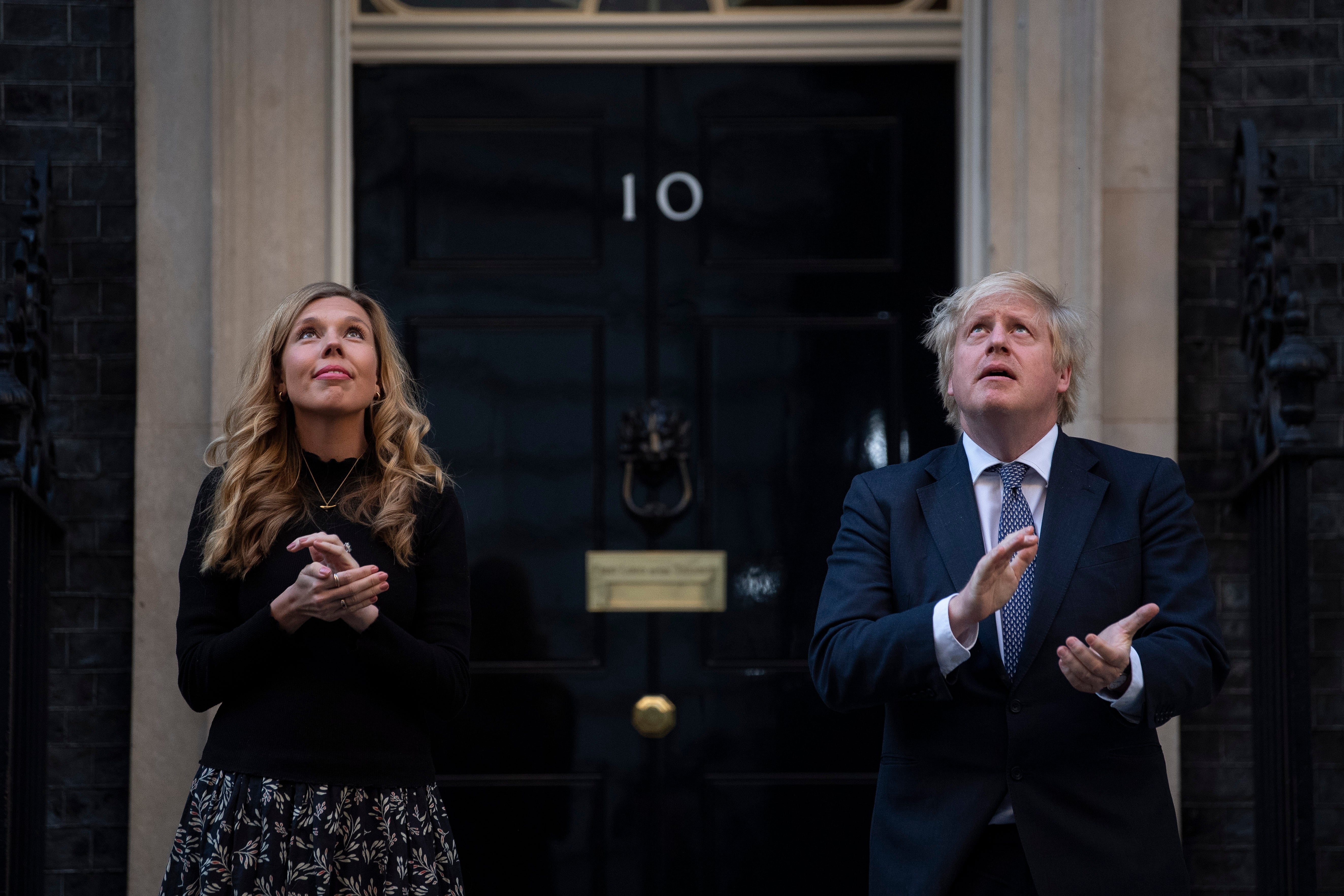This detailed photograph captures former Prime Minister of the UK, Boris Johnson, standing alongside his wife in front of the iconic 10 Downing Street. The door, prominently displaying the white number "10," is framed with white borders, featuring a large, ornate knocker and a round gold doorknob. Above the door, a gold plaque adds to the official grandeur. Boris Johnson, distinguished by his medium-long, whitish-blonde hair, is dressed in a dark blue suit paired with a white collared shirt and a blue checkered tie. His wife, with long blonde hair cascading below her shoulders, is attired in a black long-sleeve sweater and a black print skirt. Both are captured mid-clap, gazing upwards in apparent celebration, possibly in response to a significant event in the sky above, such as an airshow. The couple's joyful and uplifting mood adds a dynamic and festive tone to the historic setting.